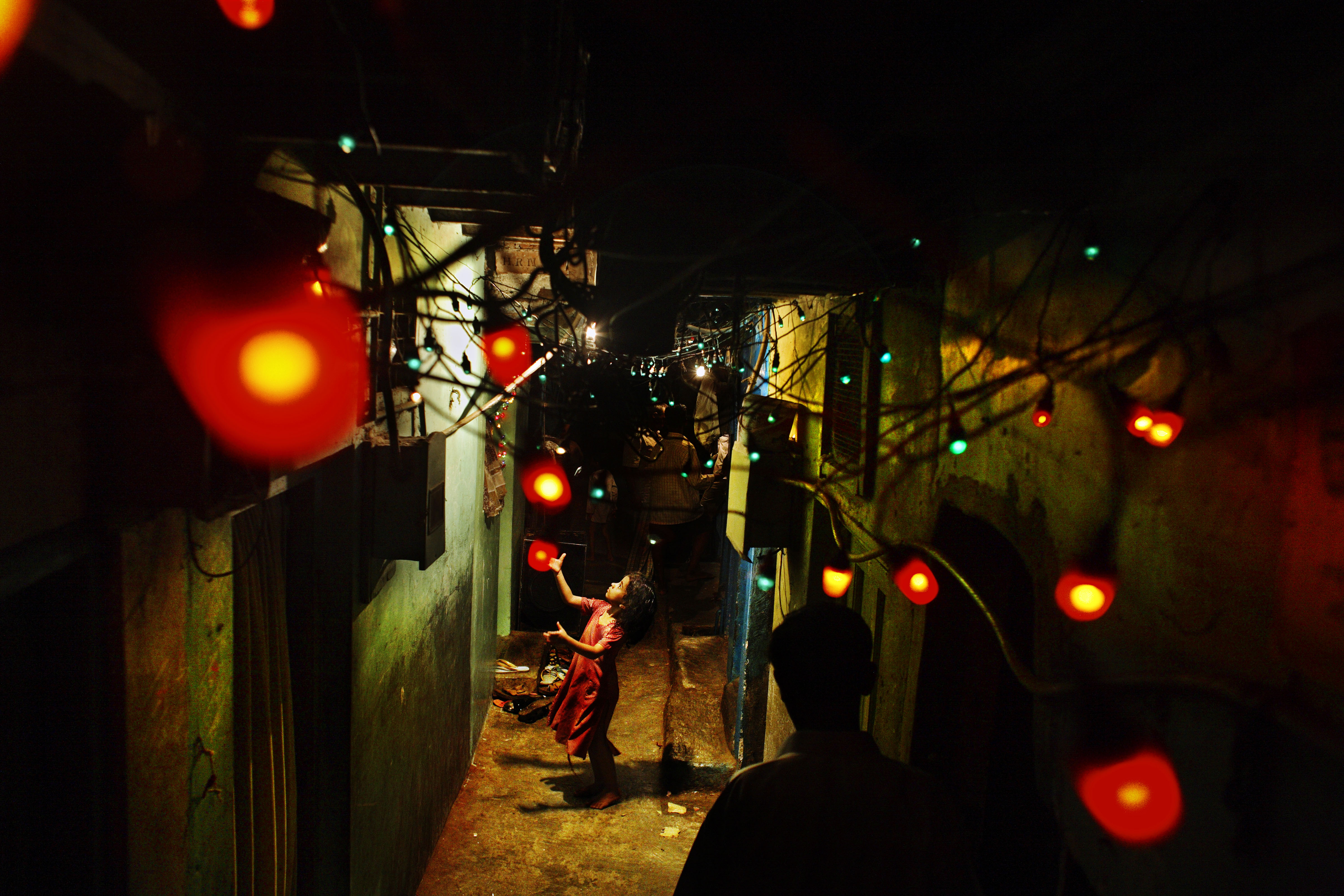In this high-quality nighttime photo, a dimly lit alleyway, possibly situated in a densely packed favela area in Brazil, stretches into blackness. The narrow passage, lined with dingy, low-income housing, is festooned with colorful lights, likely in celebration of a holiday. Red, green, and yellow bulbs are strung throughout the alley, their glow casting a festive yet somber ambiance. In the middle of the alley, about 30 feet from the camera, stands a young girl with brown hair, clad in a red dress and red shoes. She appears to be either hanging or admiring the lights, adding to the scene's charm. The alley's walls are cluttered with electrical cords, hinting at the makeshift nature of the area’s utilities. In the foreground, a shadowy male figure with a broad build and short haircut observes the girl, adding an element of mystery to the scene. Beyond her, the string of lights dwindles into the darkness, leaving the background shrouded in obscurity.